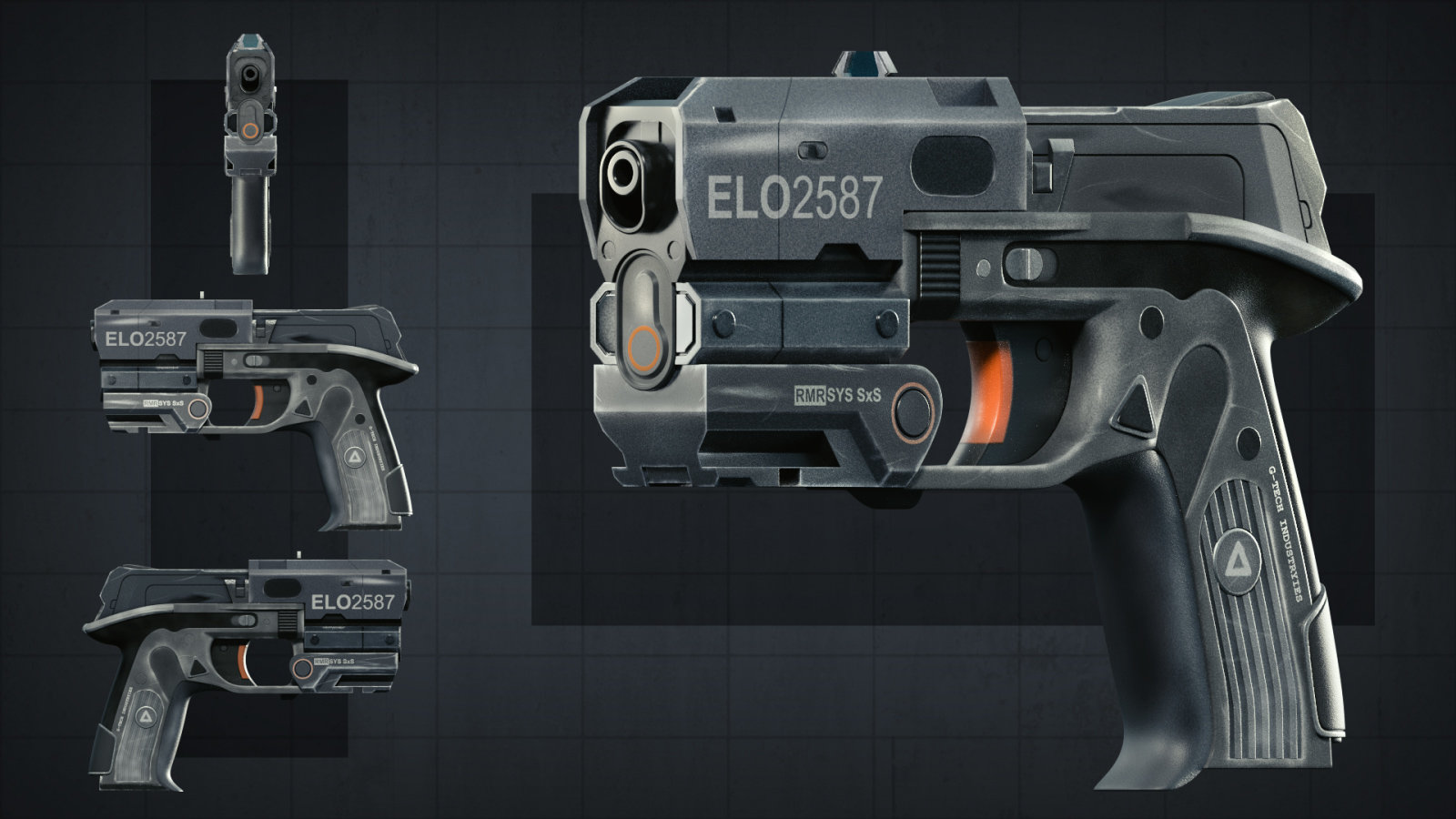The image features a detailed, possibly 3D-generated concept of a bulky, futuristic gun with the identification number "ELO2587" prominently displayed on the barrel. The gun, primarily in black and gray tones, includes an orange trigger and a small white triangle on the handle. The background is a dark gray grid, enhancing the technical aesthetic. The layout shows the weapon from multiple perspectives: a larger, slightly angled view on the right showcases the barrel pointing leftward, while smaller views on the left illustrate the gun in various orientations, including perfect profiles facing left and right. The image appears to be a design for a video game, resembling an angle sheet used in concept art.